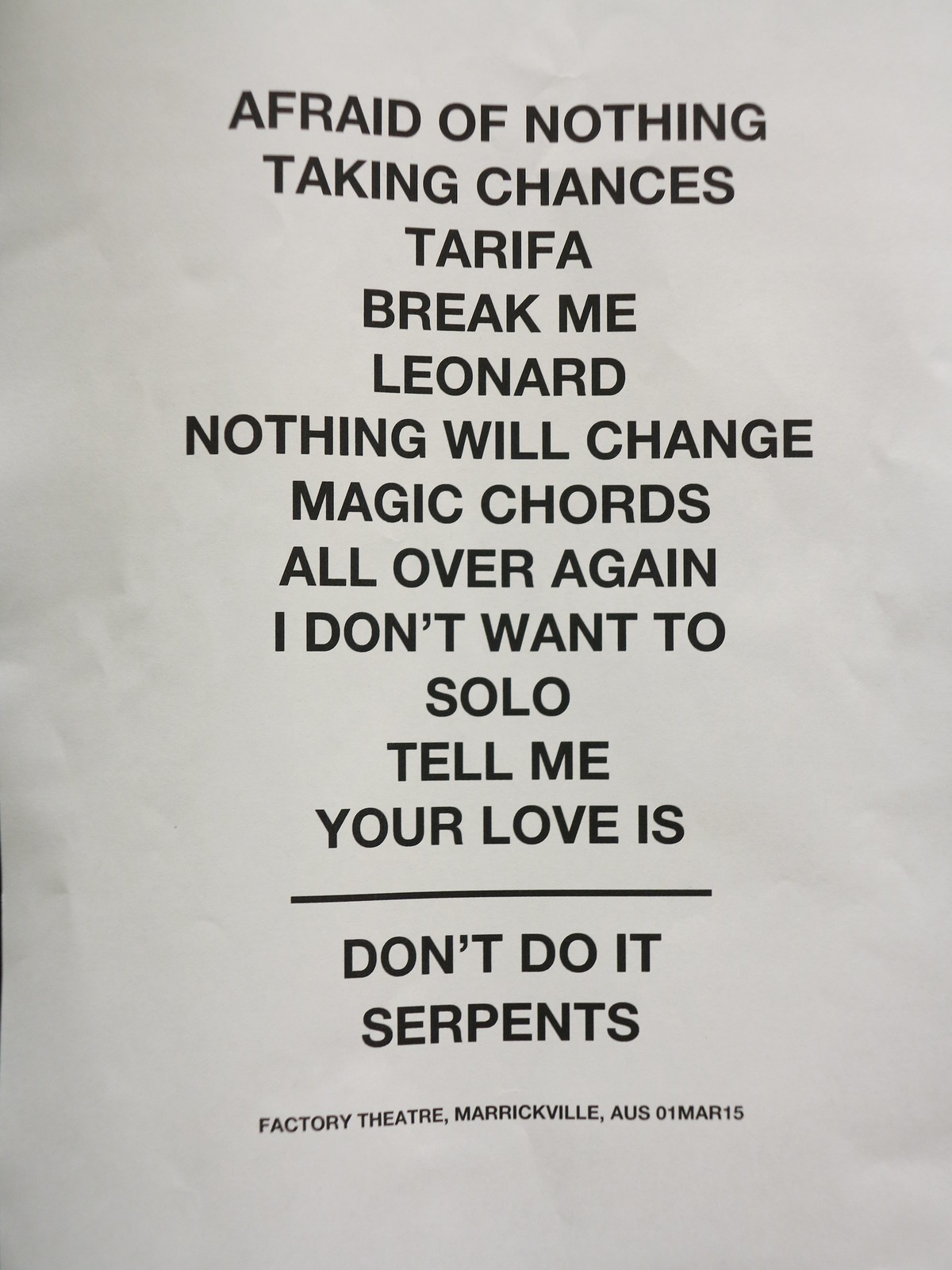The image depicts a crinkled white piece of paper with a set list printed in large, black Arial font, all in capital letters. The text is centered on the page and reads as follows: "AFRAID OF NOTHING, TAKING CHANCES, TARIFA, BREAK ME, LEONARD, NOTHING WILL CHANGE, MAGIC CHORDS, ALL OVER AGAIN, I DON'T WANT TO, SOLO, TELL ME YOUR LOVE IS." Below this, a thick black horizontal line runs the length of the phrase "YOUR LOVE IS," delineating the main set list from the encore songs. Underneath the line, the set list continues with "DON'T DO IT" and "SERPENTS." At the bottom of the page, in much smaller text, it is noted: "Factory Theater, Merrickville, AUS 01 MAR 15," indicating the venue and date of the performance.